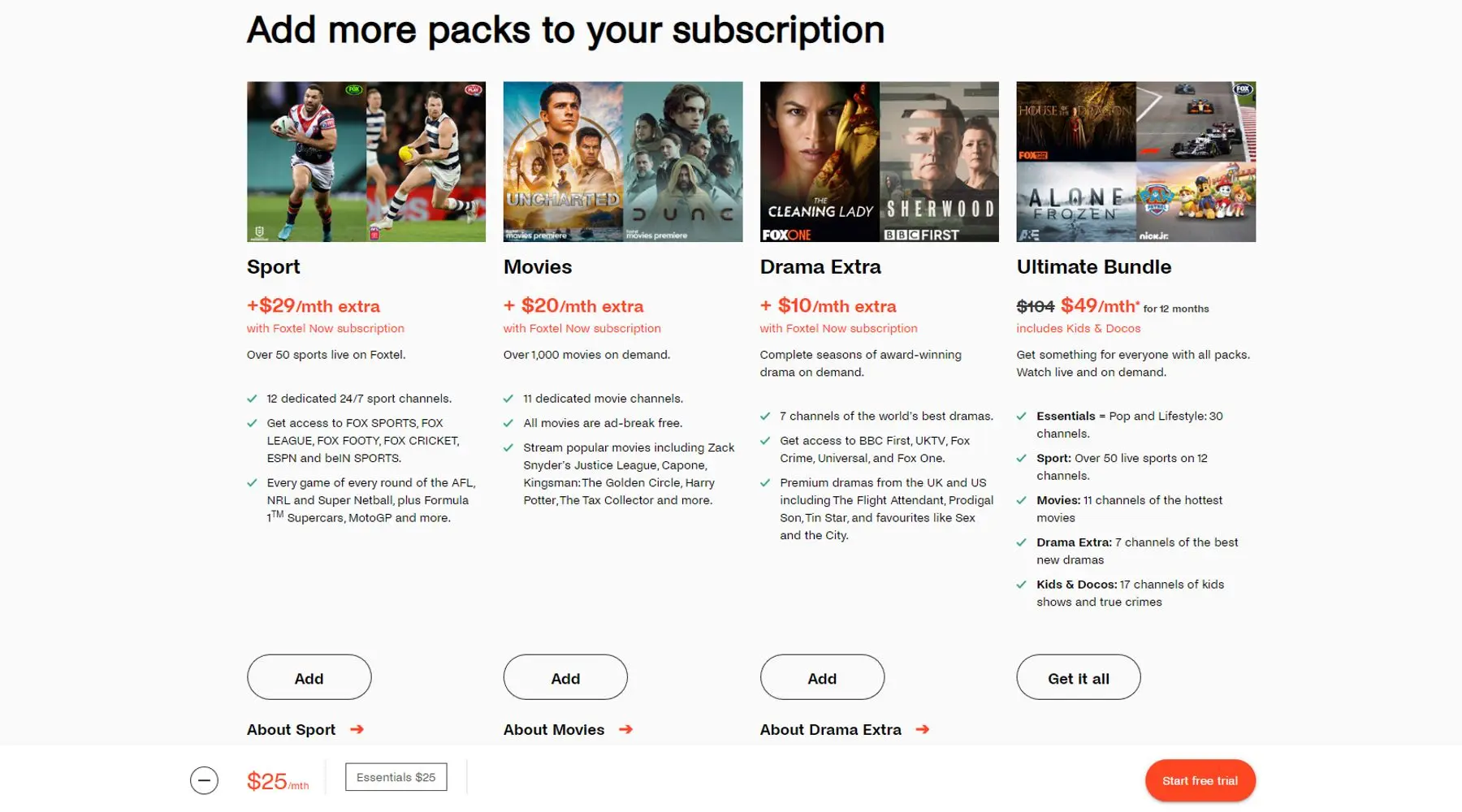The image depicts a section of an entertainment or TV service provider's website, specifically designed for adding additional packages to a subscription. The background of the webpage is a light grayish, off-white color. At the top of the page, a header in black letters reads, "Add More Packs to Your Subscription."

Below the header, on the left side, there are several options for additional packages:

1. **Sports Package**: Priced at $29 per month, this package features an image of a sports event, possibly showcasing a rugby match.
   
2. **Movies Package**: This can be added for $20 per month. The package is illustrated with images of two movies.
   
3. **Drama Extra Package**: Available for an additional $10 per month, this package includes images of two TV shows to represent its content.

4. **Ultimate Bundle**: This comprehensive package costs $50 per month and includes access to sports, movies, drama, kids' content, and essential channels.

Each package is visually represented with relevant imagery to aid in the decision-making process.